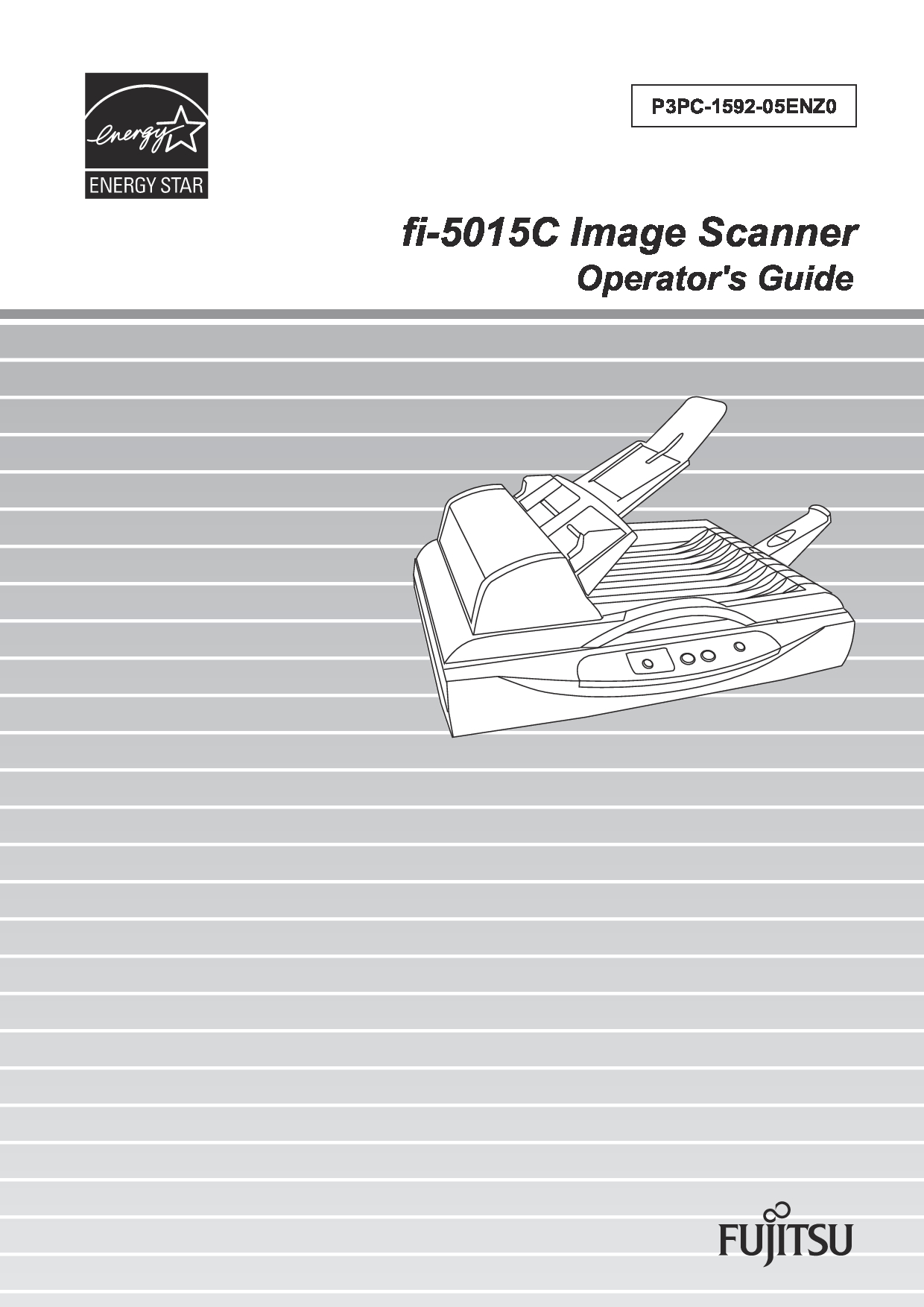The cover of the operator's guide for the Fujitsu FI-5015C image scanner prominently features a minimalist design with a white background occupying the top half. The ENERGY STAR logo, a black text on white icon signifying energy efficiency, sits in the upper left corner. Adjacent to it on the right is a code, "P3PC-1592-05ENZ0", indicating the model specification. Beneath the headline "Operator's Guide," a gray background with progressively lighter horizontal lines spans the lower half of the cover. The middle section is adorned with a line drawing of the image scanner, showing its tray and paper shoot area. The scanner has a flap on top and four side buttons. Additionally, thin gray lines run along the perimeter of the cover, and the company's name, Fujitsu, is prominently displayed at the bottom.